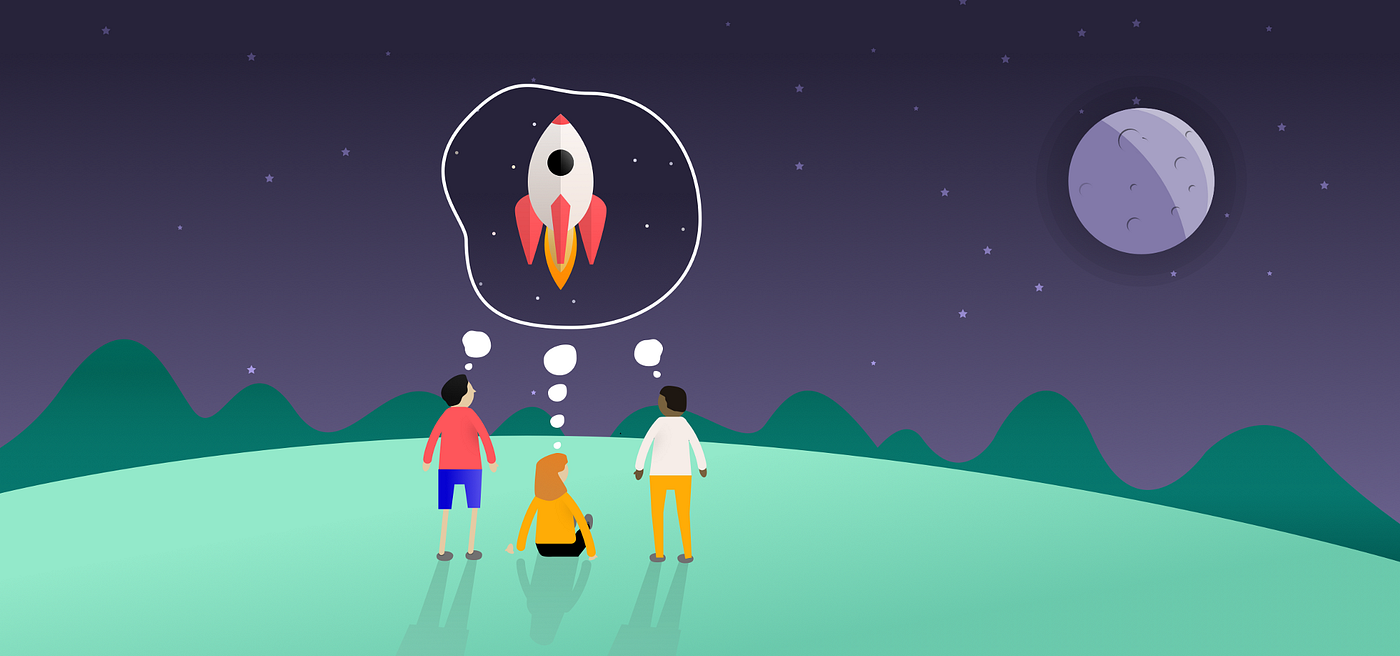The animated image showcases a serene nighttime landscape under a purplish shade of gray and black sky, dotted with white stars. The scene, stylized as a cartoon, features three people on a green hill with dark green mountains in the background. The full moon, positioned in the top right corner, is half-shadowed and half-glowing. In the center, three individuals with their backs to the viewer dream of a white spaceship. The spaceship, with a black window, red tip, three red fins, and an orange flame, is visualized through thought bubbles. The woman in the middle, sitting on the ground, wears black pants and an orange long-sleeve shirt. To her left, a man in a red long-sleeve shirt and blue shorts stands, while to her right, another man is in a white long-sleeve shirt and yellow pants. Both men have thought bubbles with two white dots, while the woman's thought bubble has four white dots, all converging into an image of the spaceship.